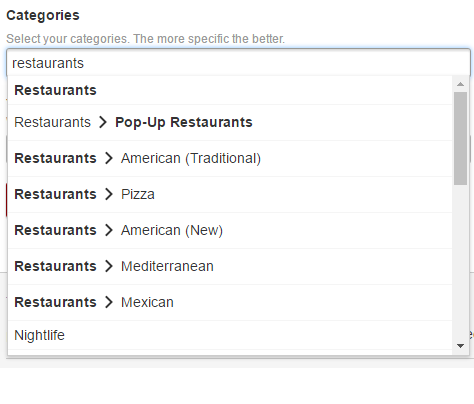The image appears to be a screenshot taken from a digital device, possibly a cell phone or computer. At the top of the screen, in bold black text, the word "Categories" is prominently displayed. Just below it, in a lighter gray text, there is a prompt: "Select your categories—the more specific the better."

The user has entered "restaurants" into a search field, triggering a list of related categories. The search results are neatly organized with the main category "Restaurants" in bold print. Each result features subcategories, following a pattern where the word "Restaurants" is accompanied by a right-pointing arrow, leading to various specific types of restaurants.

The list includes:
- "Restaurants" → "Pop Up Restaurants"
- "Restaurants" → "American (Traditional)"
- "Restaurants" → "Pizza"
- "Restaurants" → "American (New)"
- "Restaurants" → "Mediterranean"
- "Restaurants" → "Mexican"

Beneath these entries, the category "Nightlife" is also visible, potentially indicating another main category of interest.

On the far right side of the screen, a vertical search bar aligns with the content, providing users with an area to refine or enter new searches. The overall interface appears user-friendly, encouraging detailed and specific queries to better match user interests.